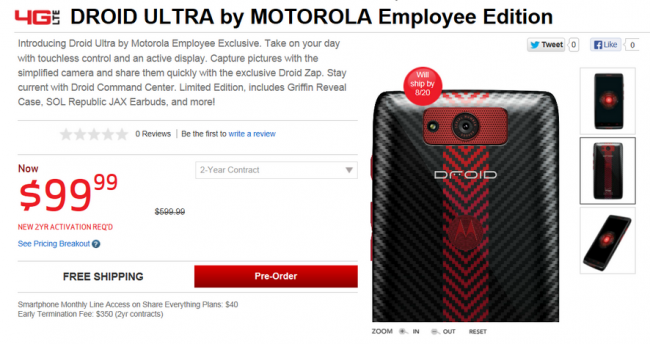Screenshot of a website displaying the Motorola Droid Ultra Employee Edition. At the top, the screen indicates 4G LTE coverage and prominently features the product name. Below, a detailed body of text describes the phone. The section includes an area for user reviews marked by stars with a note saying "0 reviews" and a prompt to "Be the first to write a review," separated by a thin line.

Directly below this review prompt, a horizontal line divides the sections. Highlighted pricing information shows "Now $9.99" in bold, with the condition "new two-year activation required" clearly mentioned underneath. Additionally, there's a blue text link for a detailed price breakdown accompanied by a blue circle with a question mark icon. To the right, the original price of $599.99 is prominently crossed out. A drop-down box offers a "two-year contract" option. Below, it states "Free Shipping" next to a bold red "Pre-order" button, supported by supplementary text that provides further details.

To the right, an image displays the front and back of the phone, showcasing its camera and black and red casing with "Droid" branding and the Motorola logo. Adjacent to the main image are three smaller thumbnail images offering different perspectives of the phone. Above the images, social media buttons for "Tweet" and "Like" are also visible.